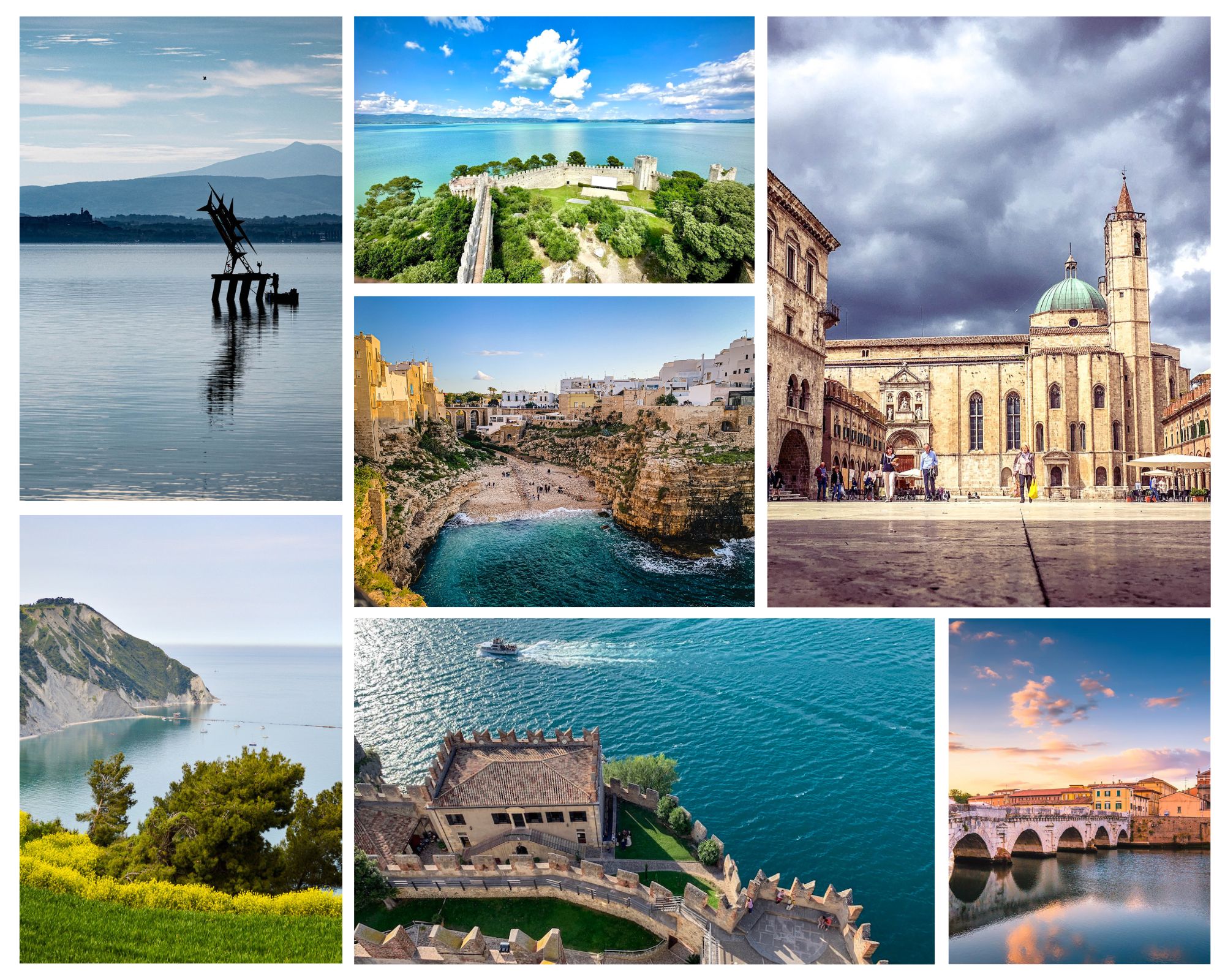This image is a compilation of seven vacation destination photographs, each capturing stunning landscapes and scenic settings, emphasizing bodies of water and historical architecture. The top left features a serene pond set against a backdrop of mountains under a blue sky. Below, in the bottom left corner, an expansive ocean view showcases vibrant blue waters with green hedges and trees in the foreground, and a mountain peeking from the left at the skyline. In the top center, an overhead shot reveals a meandering castle surrounded by lush grass, flanked by trees with the ocean and sky dotted with white clouds in the background. Below this, the center image highlights the ocean meeting the shore, bordered by ancient buildings and cliffs, framing a vast beach. The top right image, captured at ground level, displays a brown building resembling a church with a prominent tower, set against a dramatic dark sky with white clouds, with a few people visible in the courtyard. The bottom center shot takes an aerial perspective over the ocean, showing a boat navigating near the shore, where a white house with a gray rooftop is enclosed by a white fence and accessible via a curving walkway. Finally, the bottom right image presents a picturesque bridge spanning a river that leads to a distant building, all under a blue sky with fluffy clouds reflected in the water below. This collection, capturing diverse and evocative scenes, collectively underscores the allure of waterside destinations adorned with impressive structures.